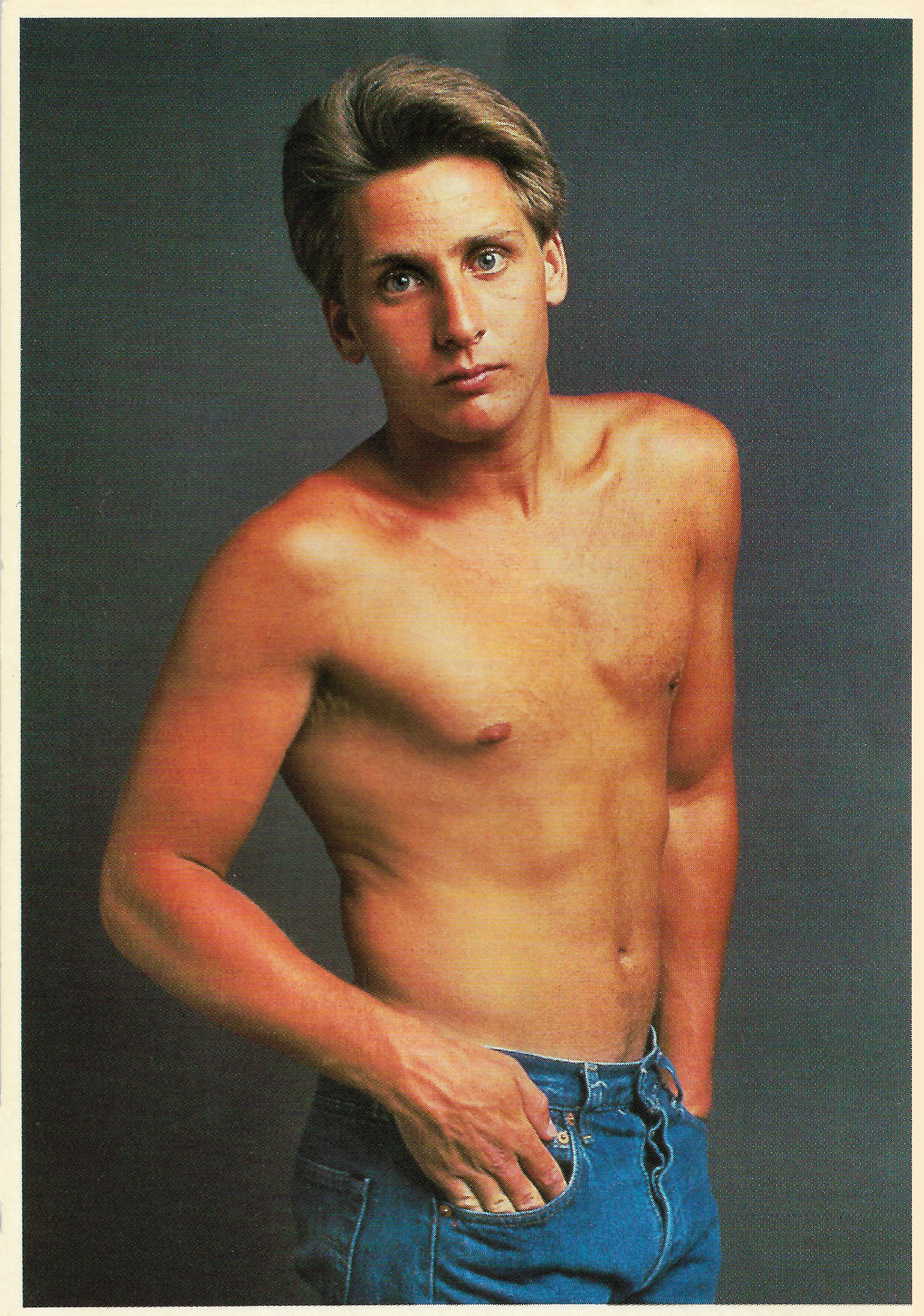This image is an old magazine scan featuring a young man who closely resembles Emilio Estevez. He stands shirtless against a dark gray background, with his hand resting slightly in the pocket of his bright blue jeans, which feature brown stitching and gold buttons but no visible brand. His blondish, feathery hair is styled up with gel, and his blue eyes gaze directly into the camera. The photo is bordered by a small white outline and contains no additional text or images, emphasizing the timeless quality of this early portrait of a now-famous actor.